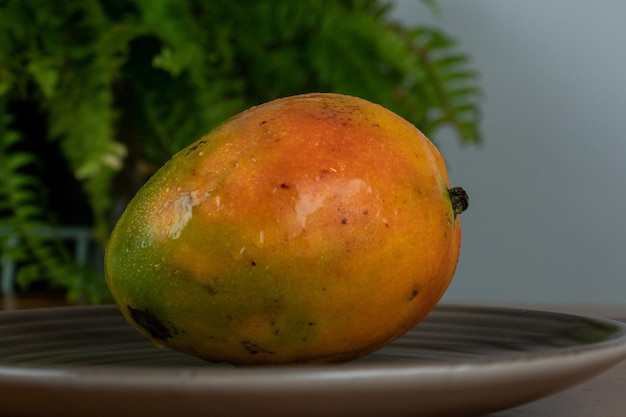The photograph features a vibrant piece of fruit, possibly a mango, resting on a round, coppery-brown ceramic plate with concentric ridges that extend to the center. The fruit is predominantly orange with hints of red, transitioning to green at the bottom, indicating it hasn't fully ripened. Black speckles and water droplets adorn its tough skin, and a small black stem peeks from the top. The plate's matte finish contrasts with the glistening fruit. In the background, an abundant green fern against a white wall adds a lush backdrop, although it remains slightly out of focus.